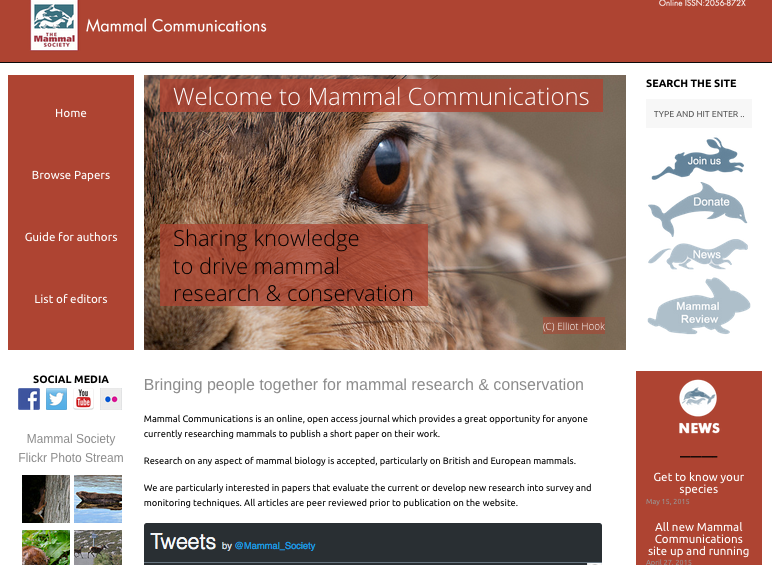Screenshot of the Mammal Communications website. The page primarily features a clean white background, accentuated with Tuscan red elements. The logo, side navigation bars, and other boxes are in this brick red color, with white text overlay.

The center of the page prominently displays a hero image with a close-up view of an animal's eye, likely a cow or a deer, showcasing detailed brown fur. Overlaid on this image, within a red box, the text reads: "Sharing knowledge to drive mammal research and conservation."

Directly below the hero image, in light gray font, it says: "Bringing people together for mammal research and conservation." The main section of the website contains text in darker black font: "Mammal Communications is an online open access journal, which provides a great opportunity for anyone currently researching mammals to publish a short paper on their work."

Side navigation bars offer links to key pages such as Home, Browse Papers, Guide for Authors, List of Editors, and more. A search box is conveniently positioned on the right side of the page, allowing users to search through the site's content.